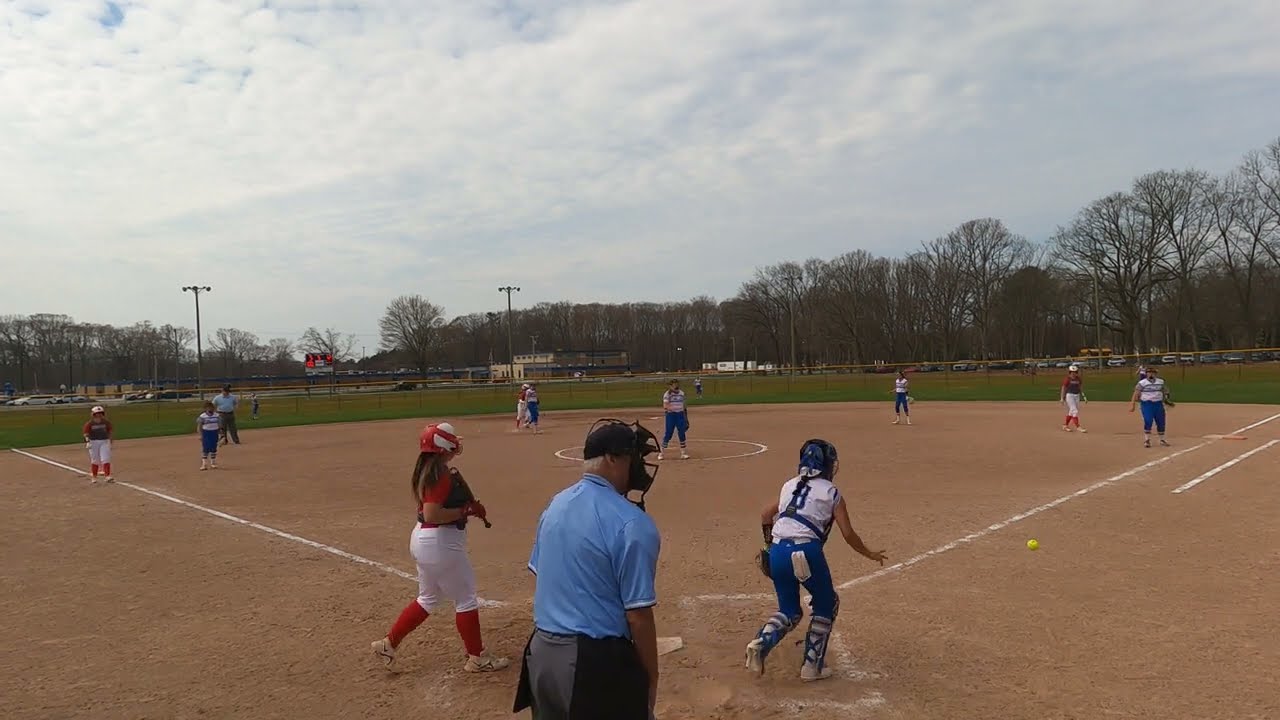In this color landscape photo taken from behind the pitcher's mound on a baseball or softball field, the central focus is the elderly Caucasian umpire dressed in a black ball cap, face mask, short-sleeved blue collared shirt, gray slacks, and an apron-like garment around his waist. The scene is bathed in daylight under a mostly cloudy sky, characterizing an overcast day. The umpire stands facing away from the camera, positioned centrally at the bottom of the image. Directly in front of him is a female player in red and white—a red shirt, white pants, red socks, sneakers, and a red and white cap—casually walking with her baseball bat towards the mound, indicating the game is not currently in active play. To the umpire's right is the catcher from the blue team, potentially throwing or preparing to catch a distinctive yellow ball. Surrounding them, the brown dusty dirt of the baseball diamond contrasts with the grassy green field and a short fence visible in the background. The distant background also features leafless trees and a parking lot to the left, with a scoreboard displaying red numbers and letters, enhancing the realism captured by this freeze-frame image, possibly taken from a low vantage point, indicating teenage sports players in a leisurely moment of the game.